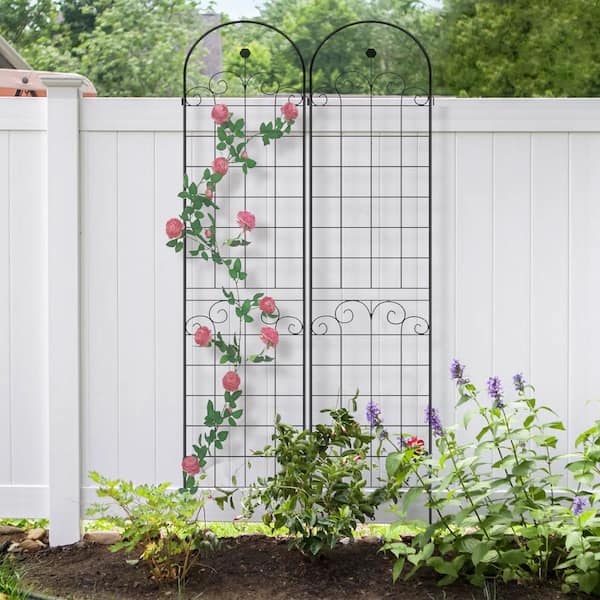This photograph, taken in a garden, features a black, metal trellis with a grid pattern and two elegantly arched tops, each adorned with a swirling design at the ends of the vertical bars. The trellis is positioned against a tall white fence, creating a striking contrast. A vibrant vine, abundant with pink roses, climbs up the left side of the trellis, intertwining gracefully through the structure for support. Below, the garden bed showcases three bushes with leafy greenery and bursts of purple flowers. Beyond the fence, tree tops are visible, adding depth to this serene garden scene.